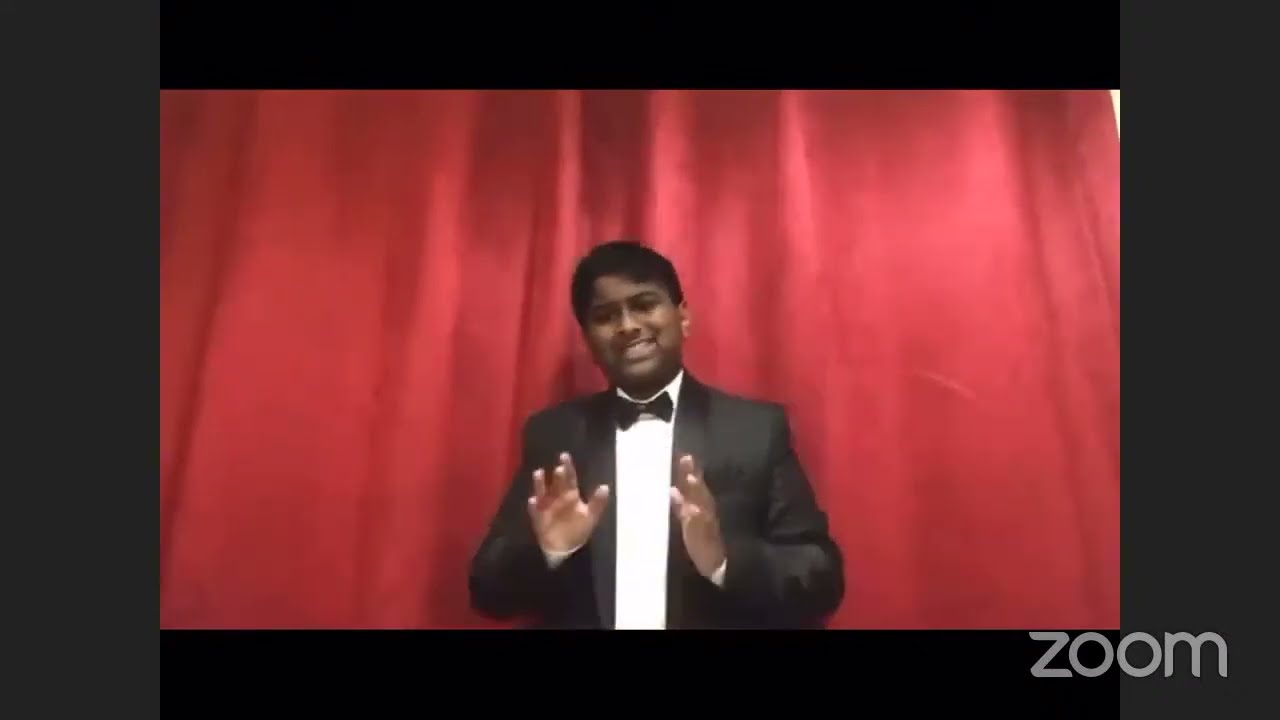This image is a still capture of a Zoom call featuring a single individual in front of a red stage curtain. The word "Zoom" appears in medium gray text in the bottom right corner, suggesting the meeting's platform. The image is framed by dark gray borders on the left and right, and black borders on the top and bottom. The person on screen is a young male, likely of Indian descent, with short black hair. He is dressed in a black and white tuxedo, including a black jacket, white shirt, and black bow tie. His head is tilted to the left, and he has a somewhat grimacing smile. His hands are raised and outstretched in front of his chest, possibly mid-gesture as if preparing to clap or emphasize a point. There are no other participants or additional text visible in the image.